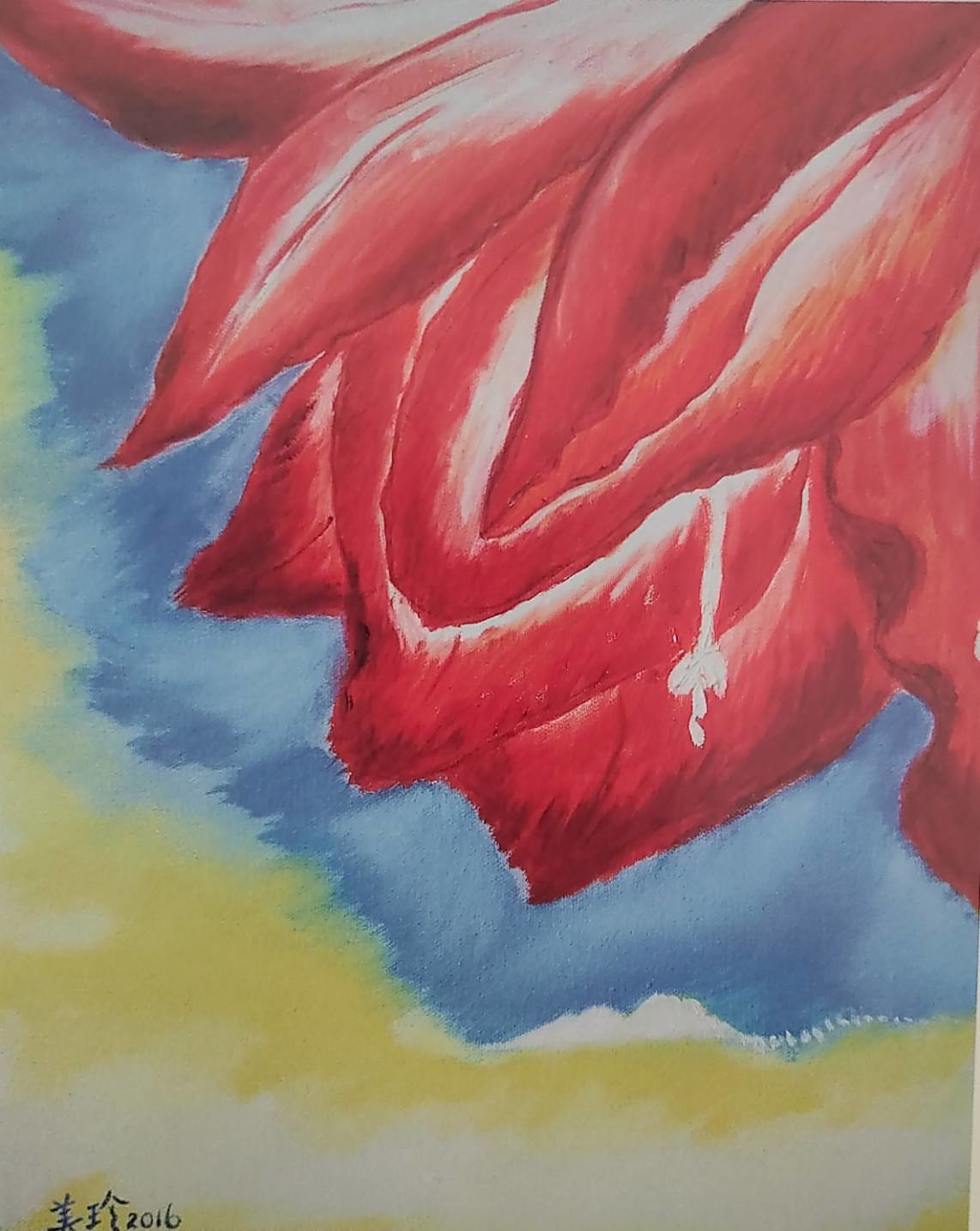A captivating watercolor painting depicting a vibrant red flower with long, elegant petals. Each petal features delicate white streaks that accentuate its three-dimensional appearance. Surrounding the flower, hues of light and dark blue are skillfully blended with touches of white and yellow, creating a visually engaging background. Notable details include the gentle curves of the petals, some arching upwards while others gracefully bend downwards. A white stem extends from the center of the flower, adding to the intricate composition. The painting is signed with Chinese or Japanese characters at the bottom, along with the year "2016" inscribed in black.